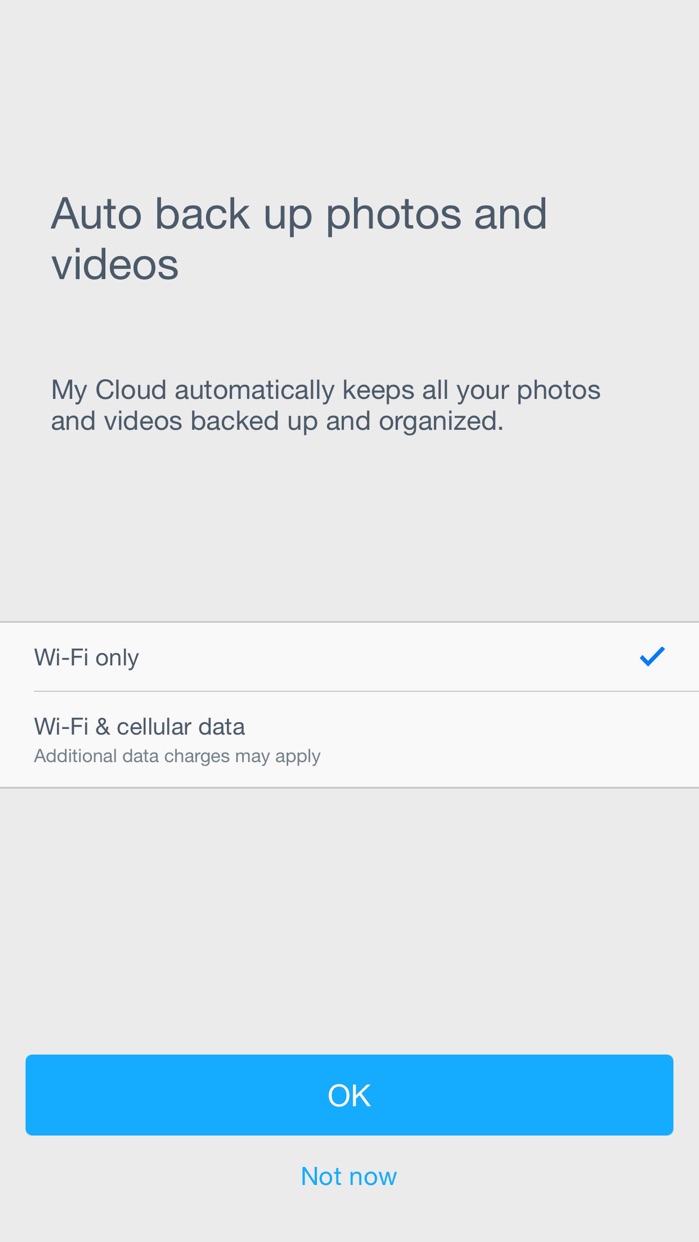The image showcases a user interface of a website designed for backing up photos and videos. The website features a dominant gray background accompanied by a dark-toned text font, creating a sleek and modern appearance. At the top of the screen, a large, bold headline states, "Auto Backup Photos and Videos," making it immediately clear what the service offers.

Beneath this headline, there is a detailed description in smaller but still noticeable font size reading, "My Cloud automatically keeps all your photos and videos backed up and organized." This implies that the service uses cloud storage to organize and store multimedia content.

Further down, the interface presents two options for data usage with checkmarks indicating selection: "Wi-Fi only" and "Wi-Fi and cellular data." A note under these options cautions, "Additional data charges may apply," highlighting potential costs for using cellular data.

The bottom portion of the interface includes a prominent blue button labeled "OK," meant to confirm user choices. Below this, in much smaller text, is an alternative option, "Not Now," for users who might not want to proceed immediately.

The overall design is classic and clean, with a user-friendly layout that is easy on the eyes, suggesting an intuitive and organized process for backing up photos and videos using a mobile device.